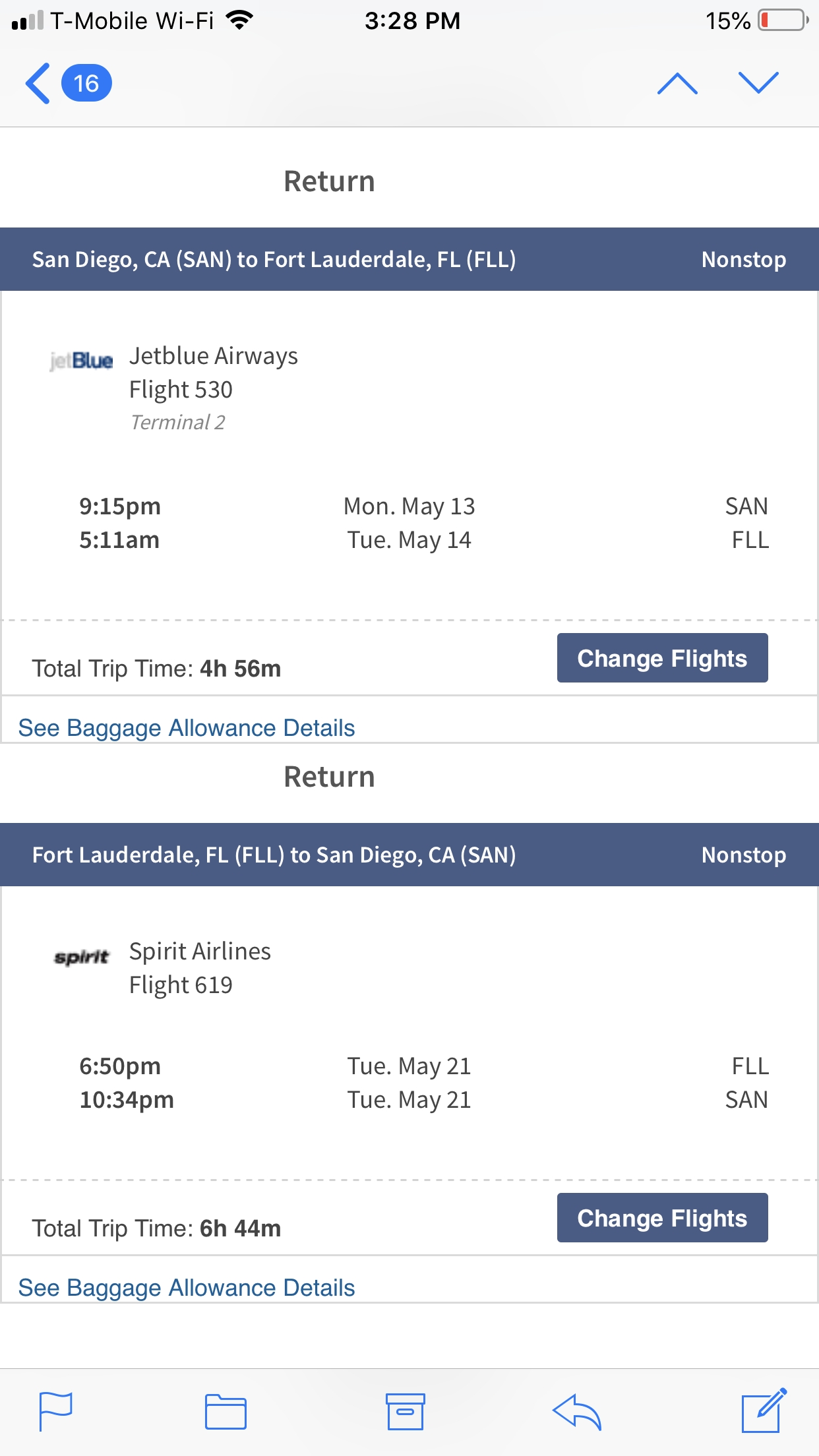The screenshot showcases a detailed flight itinerary on a mobile device with a T-Mobile carrier at 3:28 PM and 15% battery. At the top left of the screen, there is a "back" arrow encircled, followed by an up and down arrow. Here are the itinerary details:

**Outbound Flight:**
- **Route:** San Diego, CA (SAN) to Fort Lauderdale, FL (FLL)
- **Airline:** JetBlue Airways, Flight 530
- **Departure:** Terminal 2, 9:15 PM, Monday, May 13th (SAN)
- **Arrival:** 5:11 AM, Tuesday, May 14th (FLL)
- **Flight Duration:** 4 hours 56 minutes
- **Options:** 
  - A blue rectangle with "Change Flights,"
  - A hyperlink in light blue, "See Baggage Allowance Details"

**Return Flight:**
- **Route:** Fort Lauderdale, FL (FLL) to San Diego, CA (SAN)
- **Airline:** Spirit Airlines, Flight 619
- **Departure:** 6:50 PM, Tuesday, May 21st (FLL)
- **Arrival:** 10:34 PM, Tuesday, May 21st (SAN)
- **Flight Type:** Nonstop